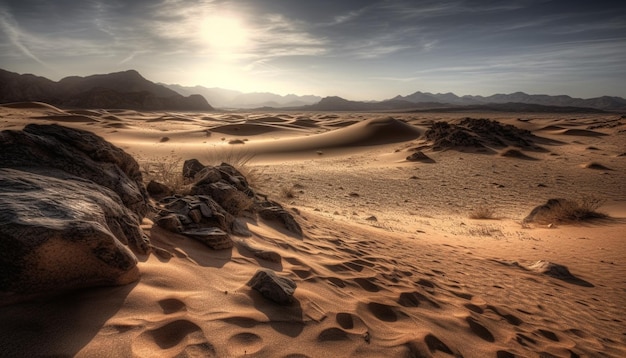This highly detailed, professional-looking image showcases a vast desert landscape under strong lighting. The terrain is predominantly sand and assorted rock formations, with some large outcroppings visible. Scattered across the foreground are numerous round footprints, possibly from an animal like a horse. The desert features relatively small dunes stretching across the scene, while distant mountains frame the horizon on both the left and right sides. The sky above is a deep blue, scattered with thin, wispy clouds that partly obscure the bright, piercing sun. Sparse patches of grass and shrubs provide minimal vegetation within this otherwise barren expanse.